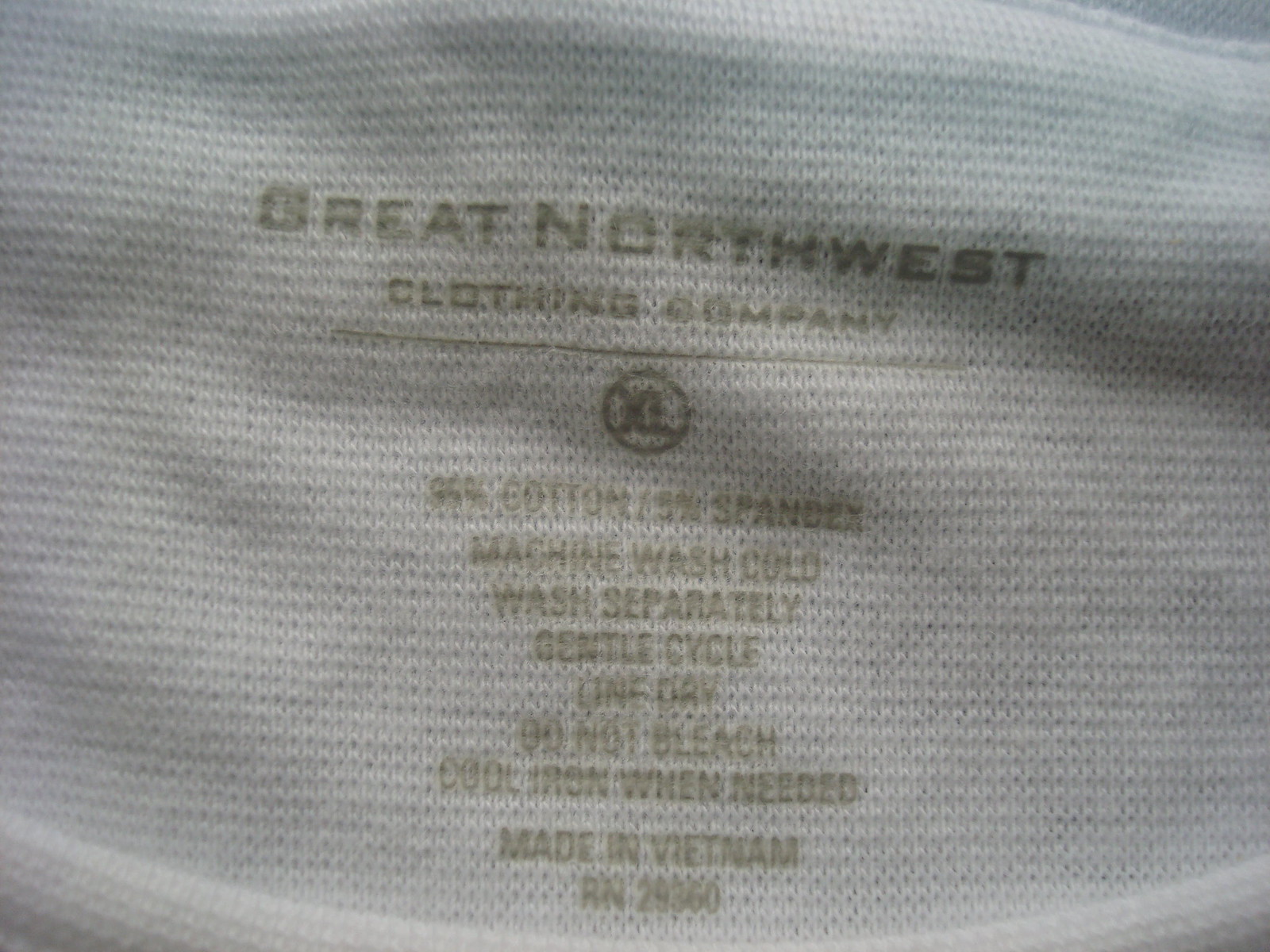This detailed close-up photograph captures the interior label of a piece of clothing, which is printed directly onto the fabric. The fabric is a white, finely textured waffle knit, and the label's text is rendered in a pea green color. At the very top of the label, in all capital letters, it reads "Great Northwest." Directly below, also centered, it states "Clothing Company." Following this, a horizontal line in the same pea green color separates the descriptors above from the sizing and care instructions below.

Centered beneath the line is a circular emblem containing the size notation "XL." The fabric composition is then listed as "34% cotton, 15% spandex." The care instructions are detailed line by line: "Machine wash cold," "Wash separately," "Gentle cycle," "Line dry," "Do not bleach," and "Cool iron when needed." At the very bottom, the label indicates the place of manufacture and a registration number, stating "Made in Vietnam," followed by "RN29960." This comprehensive and meticulously organized label ensures all necessary details about the clothing are clearly conveyed.